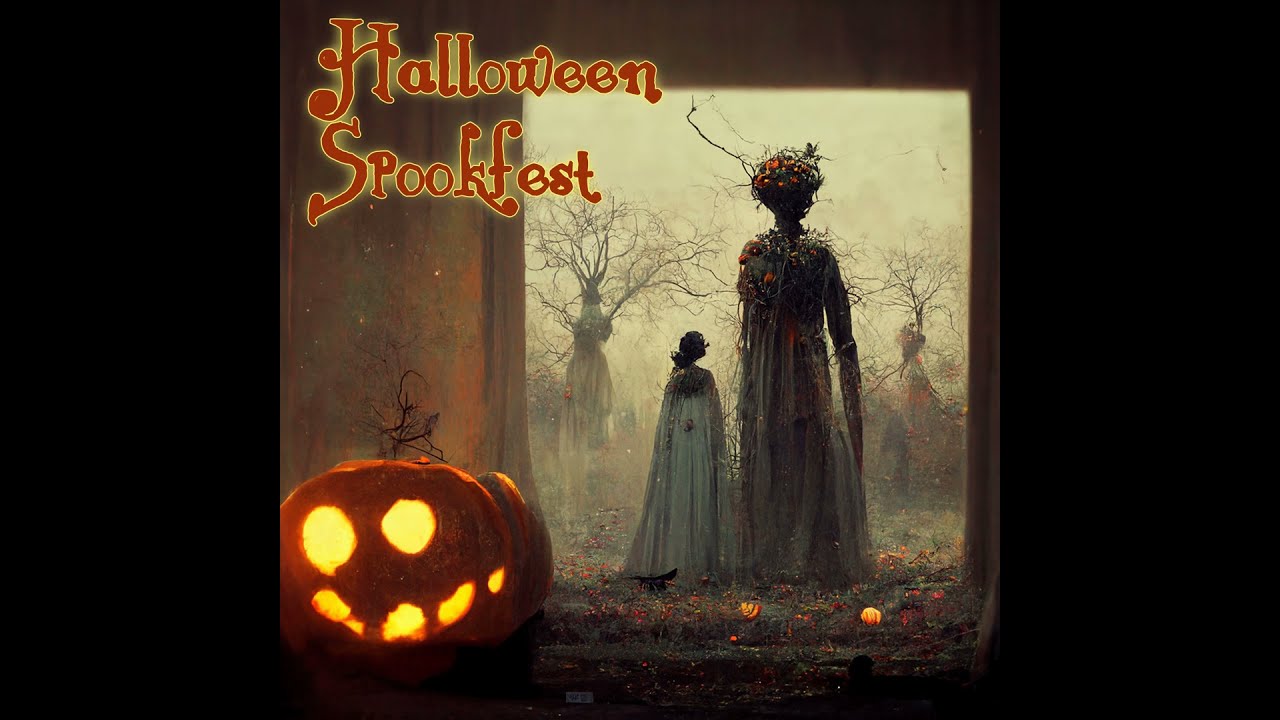The image is a hauntingly detailed poster for Halloween Spookfest, set against a stark black background. In the upper left corner, the text "Halloween Spookfest" is prominently displayed in burnt orange-red letters with a yellow-golden outline glow, adding an eerie vibe. Dominating the lower left corner is an illuminated jack-o'-lantern with two circular eyes, a mouth formed by several circles, and a small stem on top. The central focus of the image features two ethereal figures in silhouette, draped in gowns resembling wood nymphs, with flowers adorning their headdresses. They stand amidst a mystical background of tree forms, enhancing the spooky ambiance. To the right of the text, there's an impression of a doorway, hinting this scene could be set inside a barn or similar structure, adding to the overall mystery and frightful atmosphere of the poster.